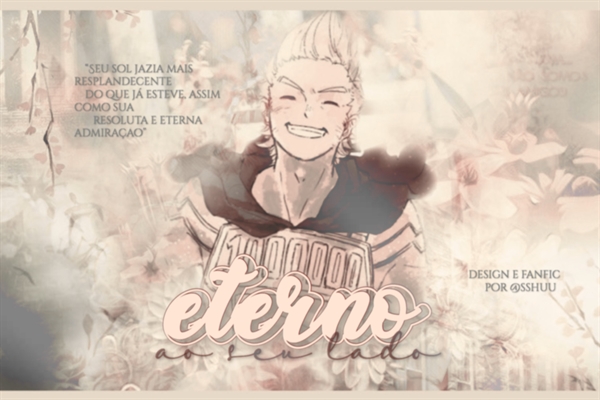The advertisement image features a semi-transparent collage of various flowers, all tinted with a pink filter that gives the entire scene a dreamy, monochromatic pink hue. Dominating the center of the image is a character from the anime "My Hero Academia," visible from the chest upwards. This character, sporting a bright, peak-swept blonde hairstyle, has an open-mouthed smile with eyes squinted shut and eyebrows pointed inward, giving him an intense yet cheerful expression. He wears a tight long-sleeve shirt and a chest plate emblazoned with the number “1000000,” with a dark-colored cape fluttering behind him. Surrounding the character, there is some text in various locations: the title "Eterno" is positioned in the upper left, while "Design e Fanfic" appears in the lower right. The color palette includes shades of pink, yellow, black, white, gray, and purple. The overall style and composition of the image give it the appearance of an anime cover or promotional material, enhanced by subtle floral accents reminiscent of cherry blossoms.